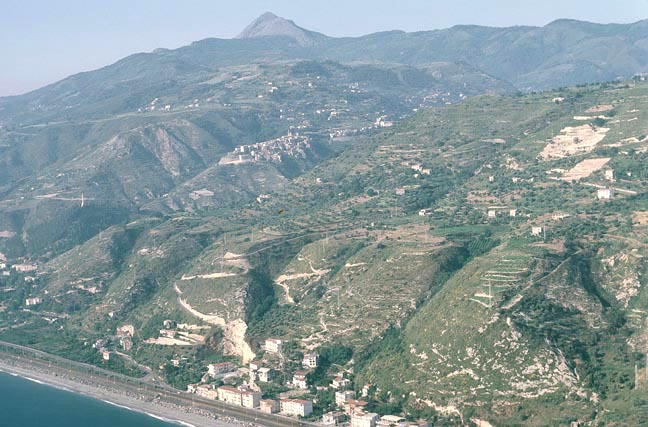The image, a drone photograph in color and landscape orientation, captures a stunning coastal and mountainous landscape. In the bottom left corner, a small portion of the deep blue ocean is visible, creating a diagonal sliver of water. Near this, a road runs from left to right, about two-thirds down the image, parallel to the coast. The lower part of the image features a quaint enclave of white houses with brown and red-tiled roofs nestled at the base of a rocky hillside. The hillsides themselves are predominantly rocky with minimal grass, though some sections reveal green patches. Scattered white sandy areas contribute to the varied texture of the terrain. Higher up the hills, scattered houses appear, particularly noticeable near the center and upper left of the image. The mountain range in the background is dark blue, reaching a prominent peak near the top middle of the image. The sky overhead is light blue, creating a serene backdrop. Overall, the photograph illustrates a harmonious blend of natural ruggedness and human habitation along a coastal hilly region.